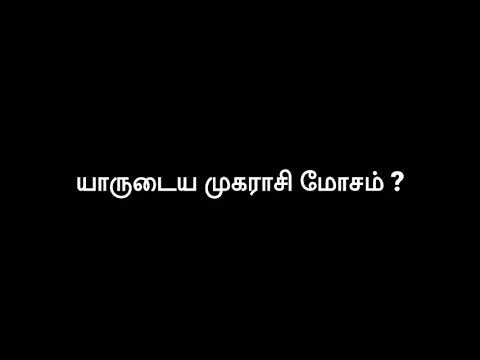The image features a solid black background with white text written in an unfamiliar script, possibly non-Western and resembling cursive or loopy characters. It is a perfect square, and the text is centered. The string of characters ends with a traditional Western question mark, distinguishing the text as a question. Despite attempts to identify the alphabet, it remains unclear, although some attempt has been made to describe individual symbols, comparing them to familiar Western letters and math symbols. The overall appearance is of a modern, stretched-out, and thin font, with certain characters featuring extensive curves and loops.